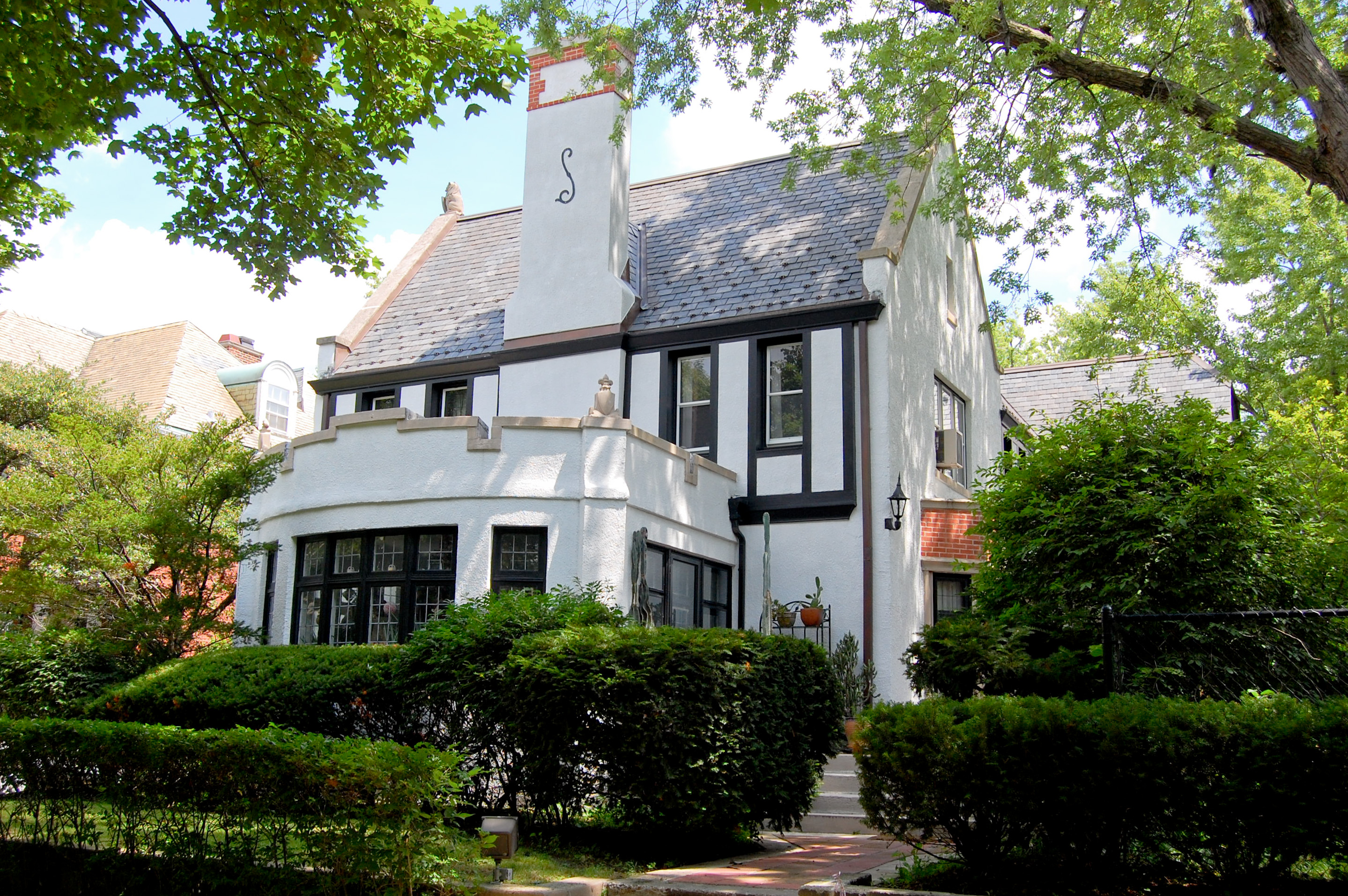This outdoor photograph captures a charming, well-maintained white house with a cottage-style aesthetic. The home features a steeply angled, tiled roof with a centrally-placed chimney that serves both the main structure and a smaller, protruding room. This chimney, primarily white with a red brick top, is adorned with a cursive 'S' in the center. Surrounding the house are neatly trimmed green bushes, with one in need of a slight trim. A brick walkway on the right side of the house leads to a set of steps, adjacent to which an old-style light fixture is mounted. The photo, taken during the daytime, showcases overhanging trees and hedgerows lining the walkway, adding to the upscale appearance of the cottage. In the right foreground, a black chain-link fence marks the edge of the property, though it is partially out of frame.